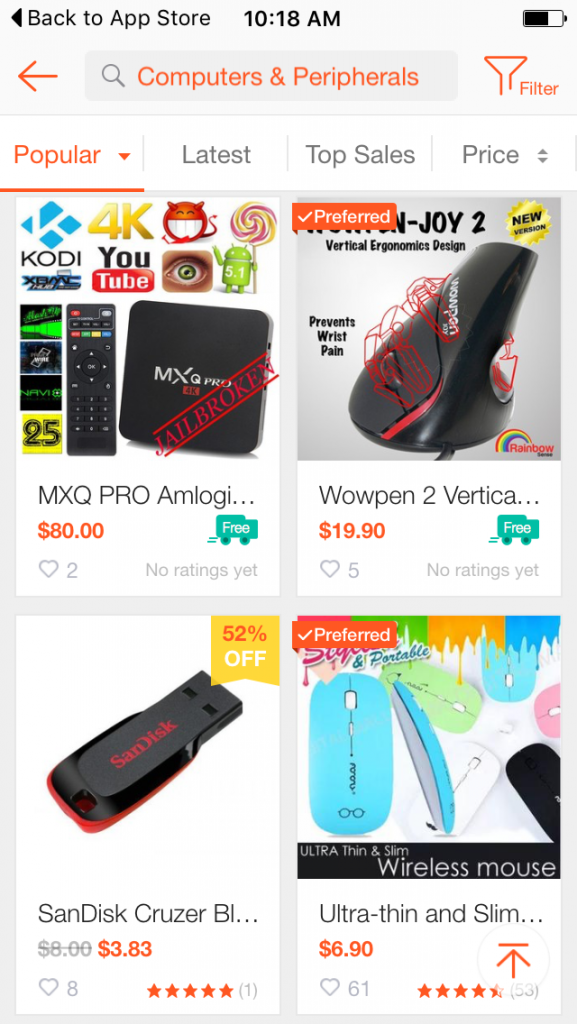In the image, a smartphone screen displays an online shop or app store interface. At the top of the screen, the search bar prominently features the text "Computer and Peripherals" in orange. To the right of the search bar is an orange filter button, while an orange back button is positioned to the left. Directly below the search bar are several tabs labeled "Popular," "Latest," "Top Sales," and "Price." The "Popular" tab is highlighted in orange, indicating it is currently selected.

Under the tabs, the first product listed is the "MXQ Pro" TV box, which supports YouTube, 4K, and Android apps. The text "Child Broken" is displayed in red, possibly indicating a product issue or status. The sleek black device is accompanied by a matching black remote control. Priced at $80 with free delivery, it has been liked by two people.

To the right of the MXQ Pro, a product called "WowPen Joy 2" is featured. This device boasts a vertical ergonomic design that helps prevent wrist pain. The black and red device is priced at $19.90 and is marked as a "Preferred" item by an orange sticker on the top right. It has been liked by five people.

In the bottom left corner of the screen, a "SanDisk Cruiser" USB drive is showcased, priced at $3.83 after a 52% discount. This highly rated USB drive has received a 5-star rating from users and is liked by eight people.

Finally, on the bottom right, an "Ultra Thin and Slim Wireless Mouse" is displayed. Available in multiple colors—blue, white, black, pink, and green—it is marked as "Preferred" with an orange sticker. The mouse costs $6.90, holds a 4.5-star rating from 53 reviews, and has been liked by 61 people. All the product prices are prominently displayed in orange.